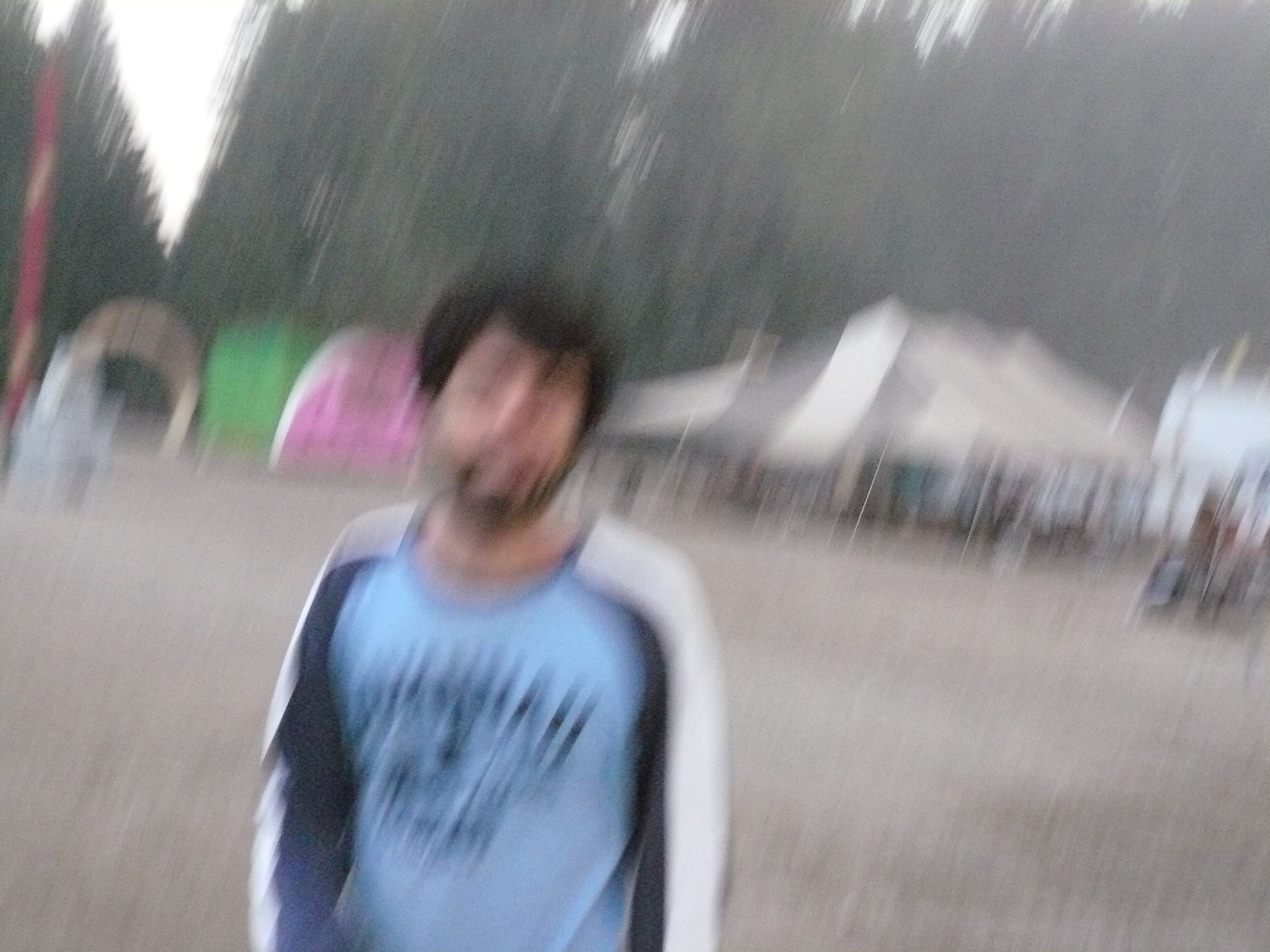The image depicts an outdoor setting featuring a man standing in front of several white tents situated on the right side of the frame. The man has black hair and sports a short mustache and beard. He is wearing a light blue shirt with white sleeves and black accents, which also has some illegible writing on it. The image is somewhat blurry, obscuring fine details of the man's face.

In the background, underneath the tents, there are indistinct figures, possibly people, adding to the bustling ambiance. To the left of the man, there's a pink object next to a green one, though their specific nature is unclear. A loop-like structure emerges from the ground near a red pole, and a garbage can is also visible.

The ground is gray and rocky, enhancing the rugged feel of the area. Behind all these elements, a dense arrangement of trees provides a natural backdrop, with the white sky peeking through in the upper left corner of the image.